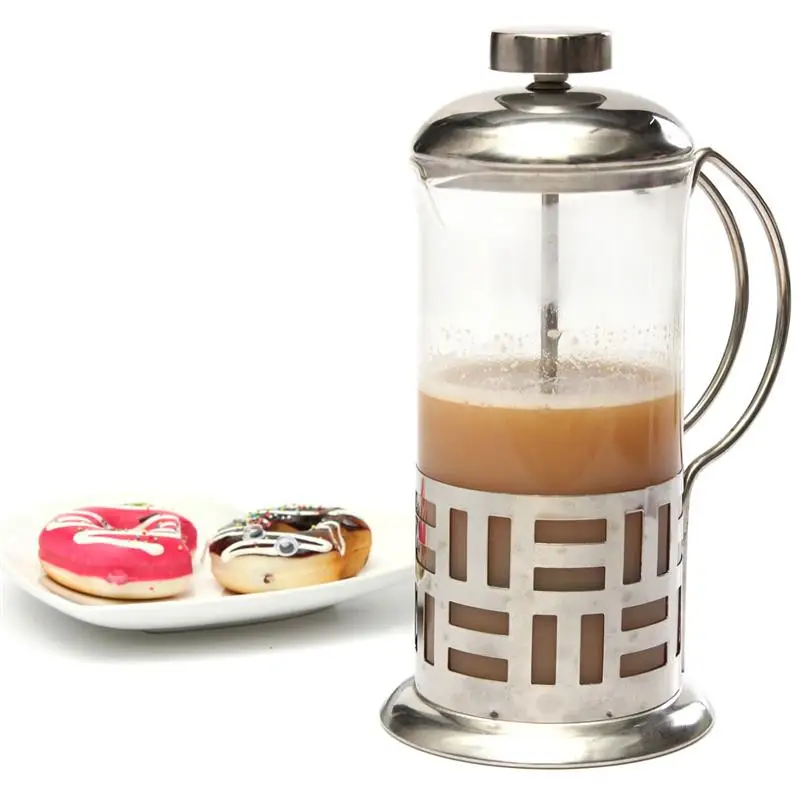The photograph displays a scene with a clean, white background, featuring a stylish coffee setup alongside a plate of doughnuts. On the right side of the image is a sophisticated cylindrical coffee maker, identified as a Bodum. The coffee maker has a distinctive design with a clear glass cylinder, half-filled with brown coffee, encased in a metallic silver frame. This frame showcases a pattern of alternating horizontal and vertical cut-out rectangles on its bottom third. The coffee maker includes a curved wire handle and is topped with a silver dome, featuring a screw cap and cylindrical rod that extends into the coffee. 

To the left of this elegant coffee device, there is a white ceramic plate with two doughnuts. The doughnut on the right is adorned with chocolate frosting, white drizzle, and sprinkled with tiny bits. The left doughnut is covered in pink frosting and also decorated with white drizzle. The entire presentation is set against a minimalist, white backdrop, emphasizing the contrast and details of the coffee and doughnuts.